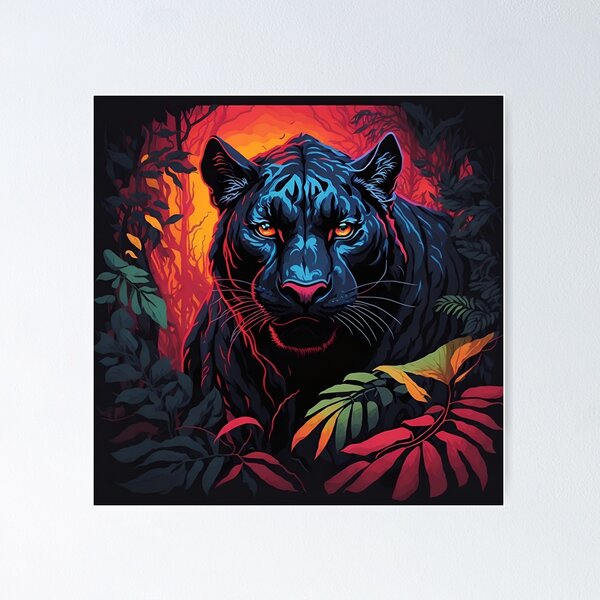This striking digital painting centers on a menacing black tiger with golden-orange eyes and a vivid pink nose, staring directly at the viewer. The tiger is uniquely colored with light blue stripes and red highlights, blending with the eerie red and orange-hued background. The foreground is lush with vibrant jungle plants, featuring an array of pink, orange, and green leaves, as well as darker green foliage in the shadows. The tiger, taking up about 75% of the frame, is illuminated by an orange glow that enhances the surreal atmosphere, suggesting a sunset setting behind it and casting a red shadow. The background also includes silhouettes of trees and branches, adding depth to the scene. The image is a dramatic and stylized illustration that contrasts dark and vibrant tones.